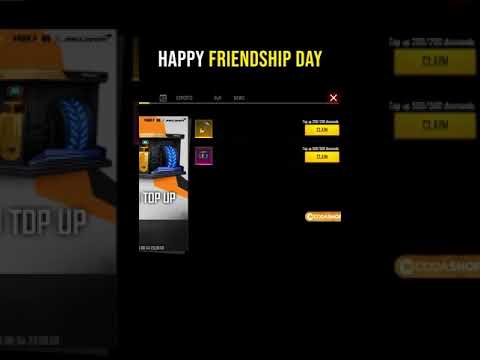The image appears to be a dark, screenshot-like representation of a computer or social media screen, primarily serving as an advertisement for Friendship Day. Centrally located, bold text reading "HAPPY FRIENDSHIP DAY" stands out, with the word "HAPPY" in white and "FRIENDSHIP DAY" in yellow, both in all capital letters. The background is black, making the text pop. On the left side of the screen, there's a vertical white rectangle with orange and blue machinery, labeled "Top Up" in white. To the right, there are bright yellow buttons labeled "Claim" and a red 'X' at the top right corner, indicating an option to close the advertisement. The image seems to repeat in a shadowed or darkened form on the right side, emphasizing the layered and mirrored layout. The overall design suggests it is an online advertisement page, potentially offering items or services for Friendship Day.